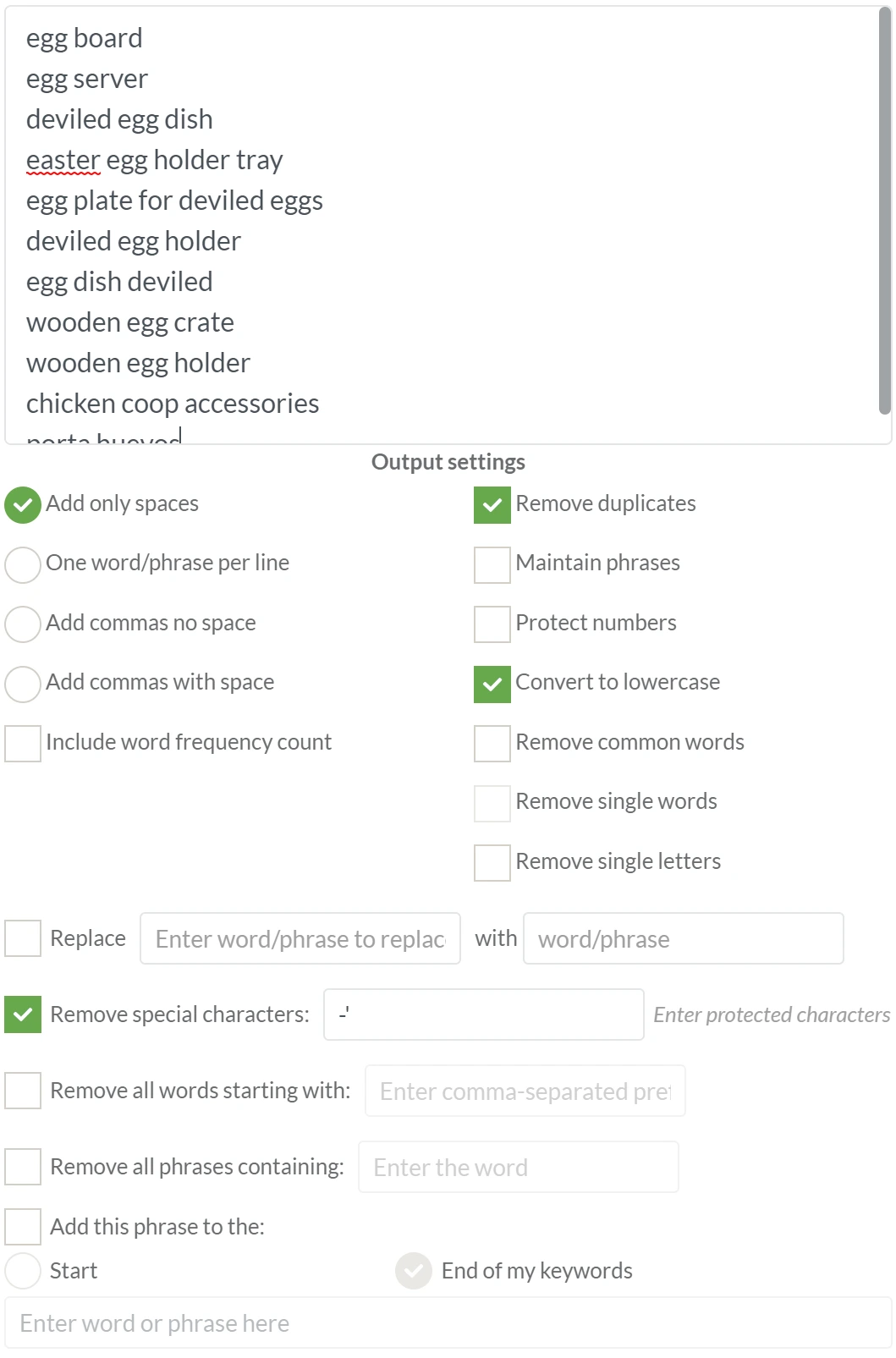**Image Description:**

The image depicts a search area interface with a variety of user input options and settings. The interface layout starts on the left, where several searched phrases are displayed prominently. These phrases include "egg board," "egg server," "deviled egg dish," "Easter egg holder tray," and "egg plate for deviled eggs." Noteworthy, the word "Easter" is underlined in red, indicating it may be a keyword or a popular search term. Additional phrases listed are "deviled egg holder," "egg dish deviled," "wooden egg crate," "wooden egg holder," and "chicken coop accessories."

To the right of the search phrases, there are settings categorized under "Output Settings." Each option has a green check mark indicating they are enabled. These settings include:
- Add only spaces
- Remove duplicates
- Convert to lowercase
- Remove special characters

Below these options, there are additional settings boxes with instructions to remove words or phrases based on specific criteria:
- "Remove all words starting with" followed by an empty input box.
- "Remove all phrases containing" followed by another empty input box.

Further down, there is another setting labelled "Add this phrase to the start," with the word "start" appearing directly beneath it.

At the bottom of the interface lies a search bar with the placeholder text "Enter word or phrase here," inviting users to input their search term.

Overall, the layout appears to be part of an advanced search or filtering tool designed for organizing and refining search results related to egg-related items and accessories.